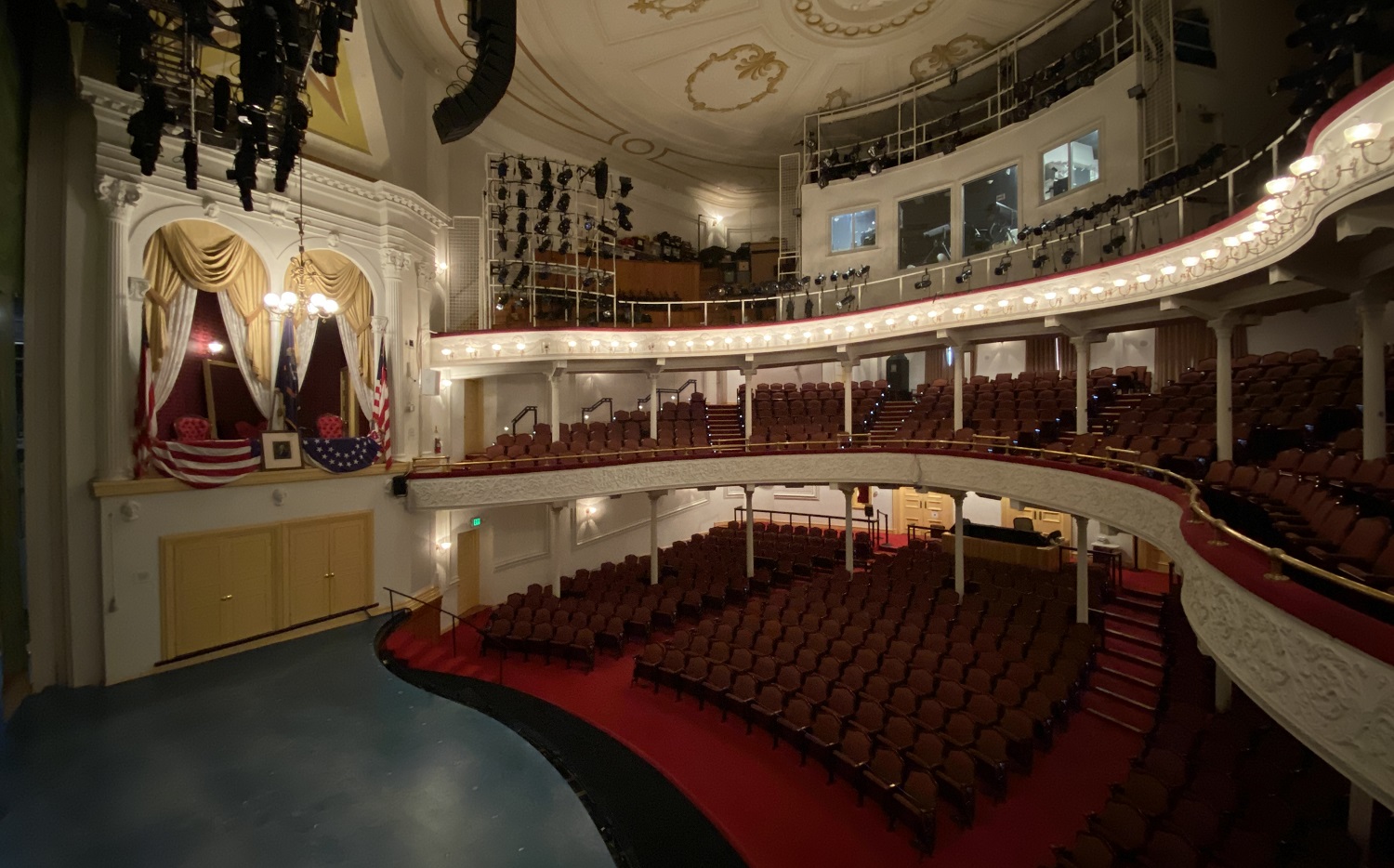The image depicts a tall and spacious auditorium with a high ceiling, viewed from an elevated position. The stage area is situated in the lower left corner, featuring a glossy, dark blue floor adjacent to black patches. Surrounding the stage, red carpeted steps descend into an aisle flanked by rows of black bleacher-style seats. These seats are divided into a smaller left section and a larger right section, both extending towards the back of the auditorium. 

White columns and beams support the structure, rising through at least two additional levels, each tier featuring further rows of seating. The second and third levels, accessible via stairs of indistinct color, maintain similar seating arrangements with white pillars. The third level seems dedicated to lighting and audio equipment rather than spectator seating, indicated by a white area with windows likely used by technical staff or a director.

In the upper left section, the auditorium showcases expensively adorned balcony seats, complete with white and gold curtains and an American flag draped nearby. Another flag is situated to the right of the stage. The ceiling is detailed with white and golden inlays, contributing to the auditorium's grandeur. Throughout the space, numerous lights ensure the area is well-illuminated, enhancing the overall visual appeal.